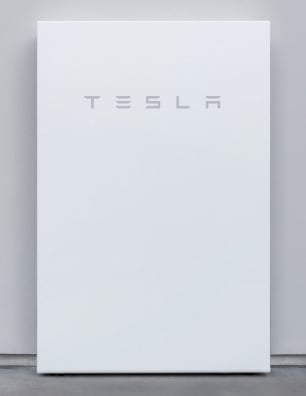The image features a tall, white, rectangular box standing upright against a white wall. The box prominently displays the Tesla logo, characterized by its unique typography. The letter "E" in "Tesla" is represented by three stacked horizontal lines, while the letter "A" features a vertical line next to a rotated bracket-like shape. The rest of the letters in the Tesla name are in a standard font. The box casts a shadow on the wall behind it, adding depth to the scene. Below the box, there is a gap between the wall and the floor, which is visible. The floor appears to be made of a gray material, possibly granite or asphalt, with the box casting a shadow on the ground.